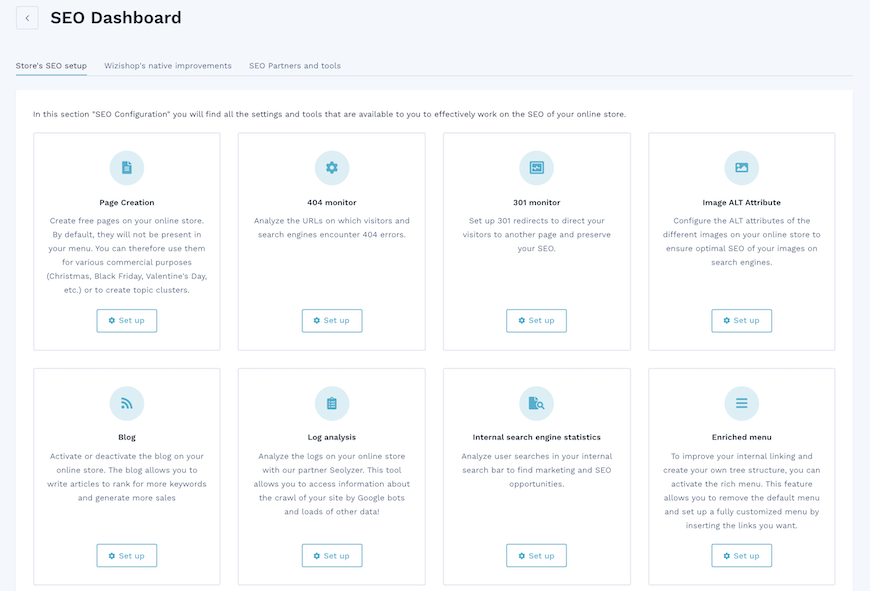The image depicts a detailed and structured SEO Dashboard, designed to assist users with managing their online store SEO effectively. At the very top, a light gray border prominently displays the title "SEO Dashboard." Directly below, a navigational menu spans horizontally, featuring the following options: Stores, SEO Setup, Workshops, Native Improvements, and SEO Partners and Tools.

Beneath this menu, the dashboard is divided into an organized grid layout on a white background, consisting of two rows with four square blocks each. A section heading reads, "SEO Configuration Get Started," indicating that users can find various settings and tools here to optimize their online store's SEO performance.

In the top row, the four blocks display the following options:
1. **Page Creation** - Includes an activation "Setup" button at the bottom.
2. **404 Monitor** - Comes with a setup button for configuration.
3. **301 Monitor** - Also equipped with a setup button for easy access.
4. **Image ALT Attribute** - Features a setup button for adjustments.

Similarly, the bottom row consists of:
1. **Blog** - Includes a setup button for integration.
2. **Blog Analysis** - Contains a setup button.
3. **Internet Search Engine Statistics** - Offers a setup button for review and analysis.
4. **Enriched Menu** - Equipped with a setup button for enhancements.

Each of these options is accompanied by a concise descriptive paragraph, detailing its functionality and importance. Icons are placed above each title, providing a visual aid to quickly identify the different sections.